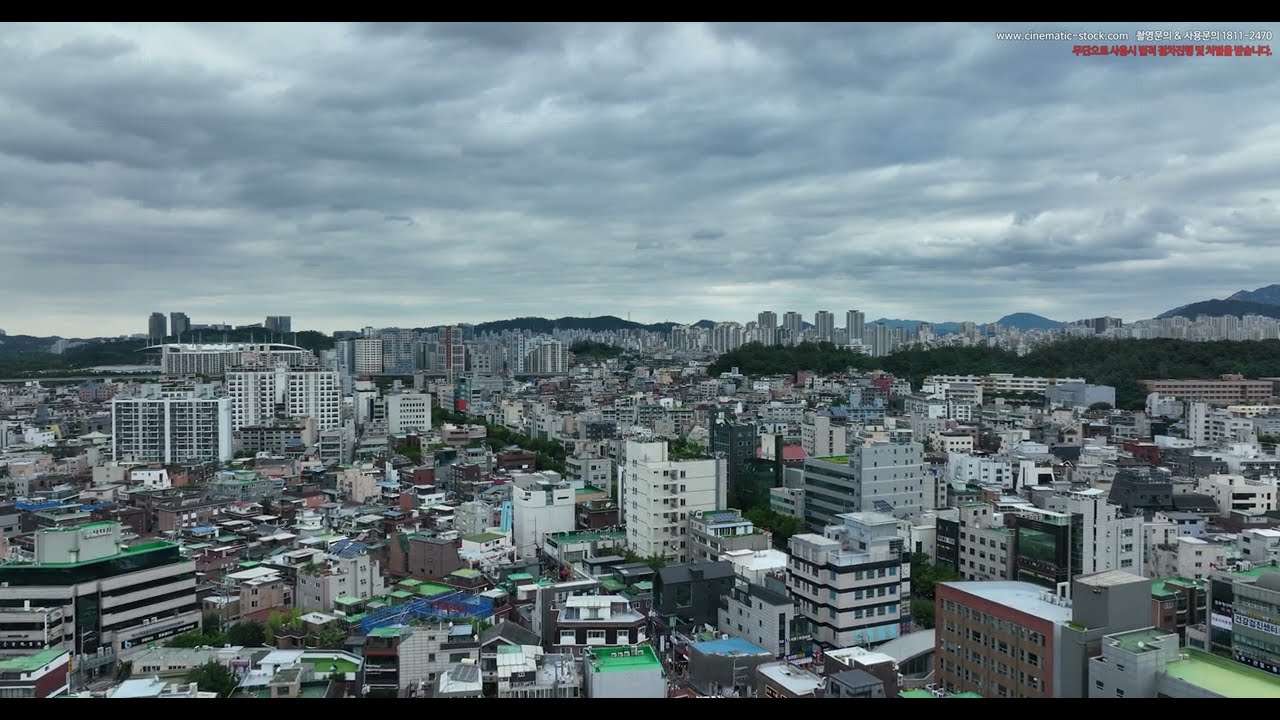The image captures a detailed and elevated view over a densely populated urban city, taken from about 100 feet above ground. The camera looks directly forward across the city's landscape, with the horizon positioned about halfway up the frame and bordered by slight mountains in the distance. Above the city, a very cloudy sky dominates the upper half. Skyscrapers scatter throughout, though none are particularly spectacular, with most buildings ranging from 10 to 20 stories tall. Many rooftops, especially those in the foreground, are painted green and blue, adding a splash of color to the otherwise dense metropolitan environment. In the upper right-hand corner, white text prominently displays the website "www.cinema-dot.com" alongside Korean characters, followed by the number "1811-2470". Beneath this white text, additional Korean or possibly mixed Chinese characters are written in red.